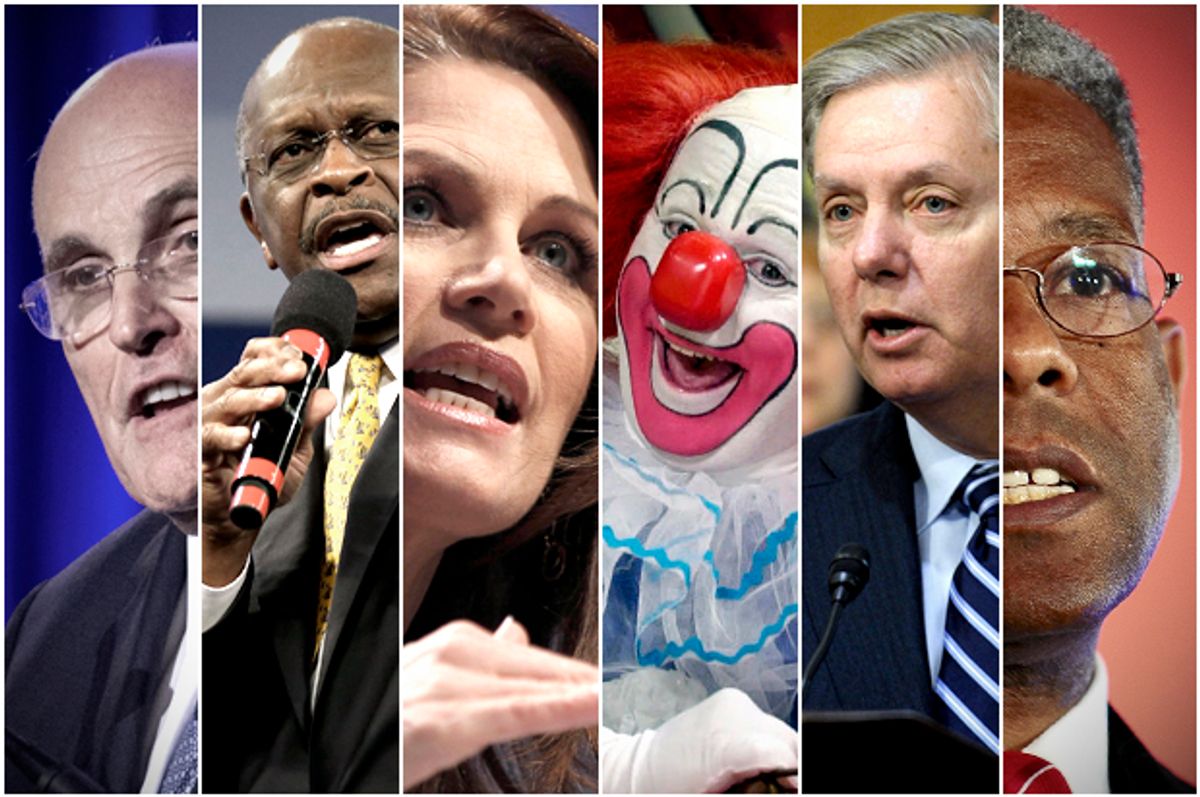The image is a large, rectangular collage featuring six distinct color photographs, separated by white vertical lines. Each photo showcases a different individual, primarily in professional settings. From left to right, the first image partially shows Rudy Giuliani, followed by a partial image of Herman Cain speaking into a microphone. The third image is of Christy Ngo, gesturing with her right hand. The fourth image stands out with Bozo the Clown, complete with a red wig, white face paint, bright red nose, a big smile, and a white ruff accented with blue detailing. Next is Senator Lindsey Graham, speaking at a podium. The final image depicts an African American man with round eyeglasses, short gray and black hair, wearing a white shirt, a red tie, and a black jacket. The collage predominantly features individuals who appear to be politicians or public figures, dressed in formal attire and engaged in speech, underscoring their professional and prominent statuses. The inclusion of the clown amidst the otherwise serious figures adds a stark and striking visual contrast.